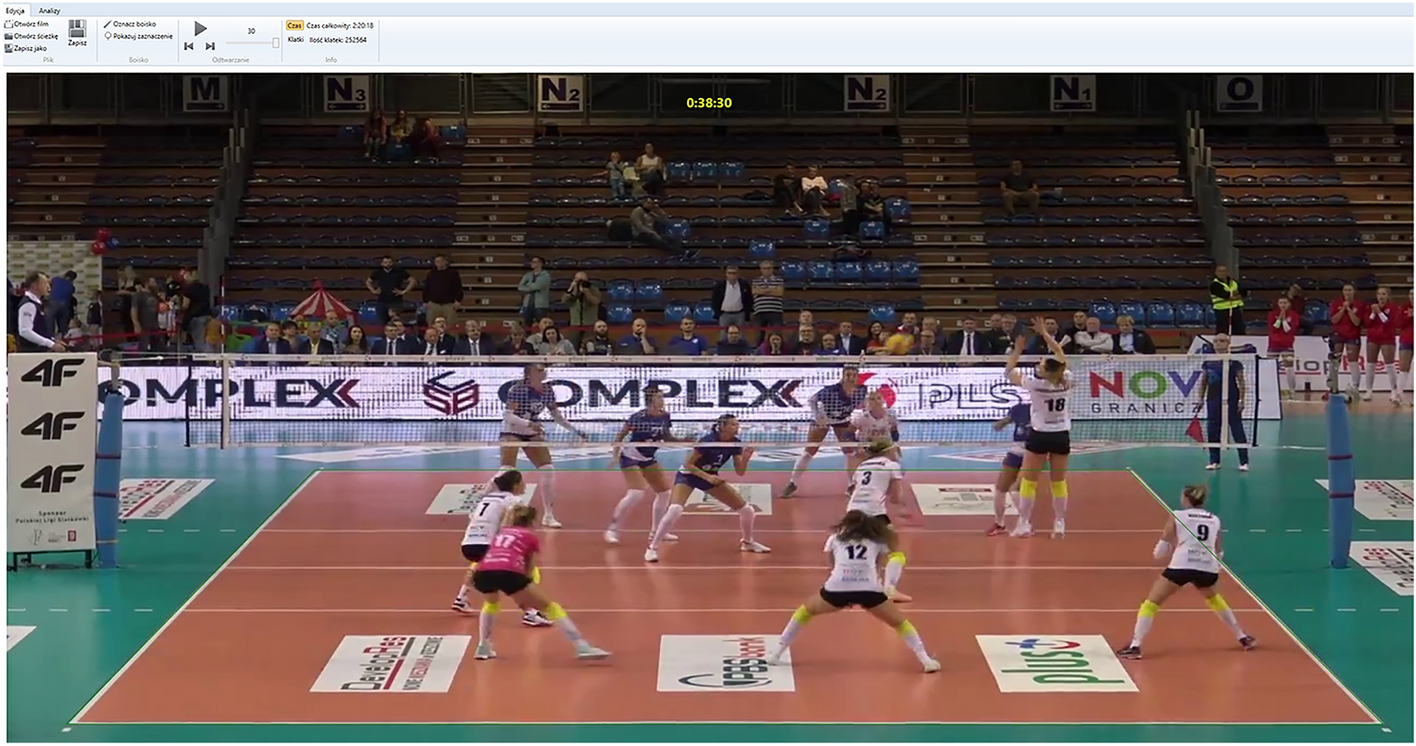This indoor color photograph captures an action-packed moment in a women's volleyball game, played on an orange court featuring logos and surrounded by a green gymnasium floor. The nearest team to the camera wears white shirts, black shorts, white socks, and yellow knee protectors, except for one player on the left in a pink jersey. Visible players include numbers 1, 3, 9, 12, 17, and 18, who is mid-jump. The opposing team don blue tops, blue shorts, and white knee protectors. The game unfolds beneath a taut net, with the ball's exact location indeterminate.

In the background, the playing area is framed by a barrier and stadium seating, which extends around 15-20 rows deep, mostly occupied in the first few rows. To the far left, a small booth marked “4F” several times houses another official, and a large sign reads "complex." A few people can be seen in reflective vests, suits, and red outfits, possibly indicating team members or staff. The top of the image reveals part of a digital clock displaying "3830" and interfaces from a video playback program, including play, advance, reverse, and save icons, hinting the photo might be a captured still from a video.